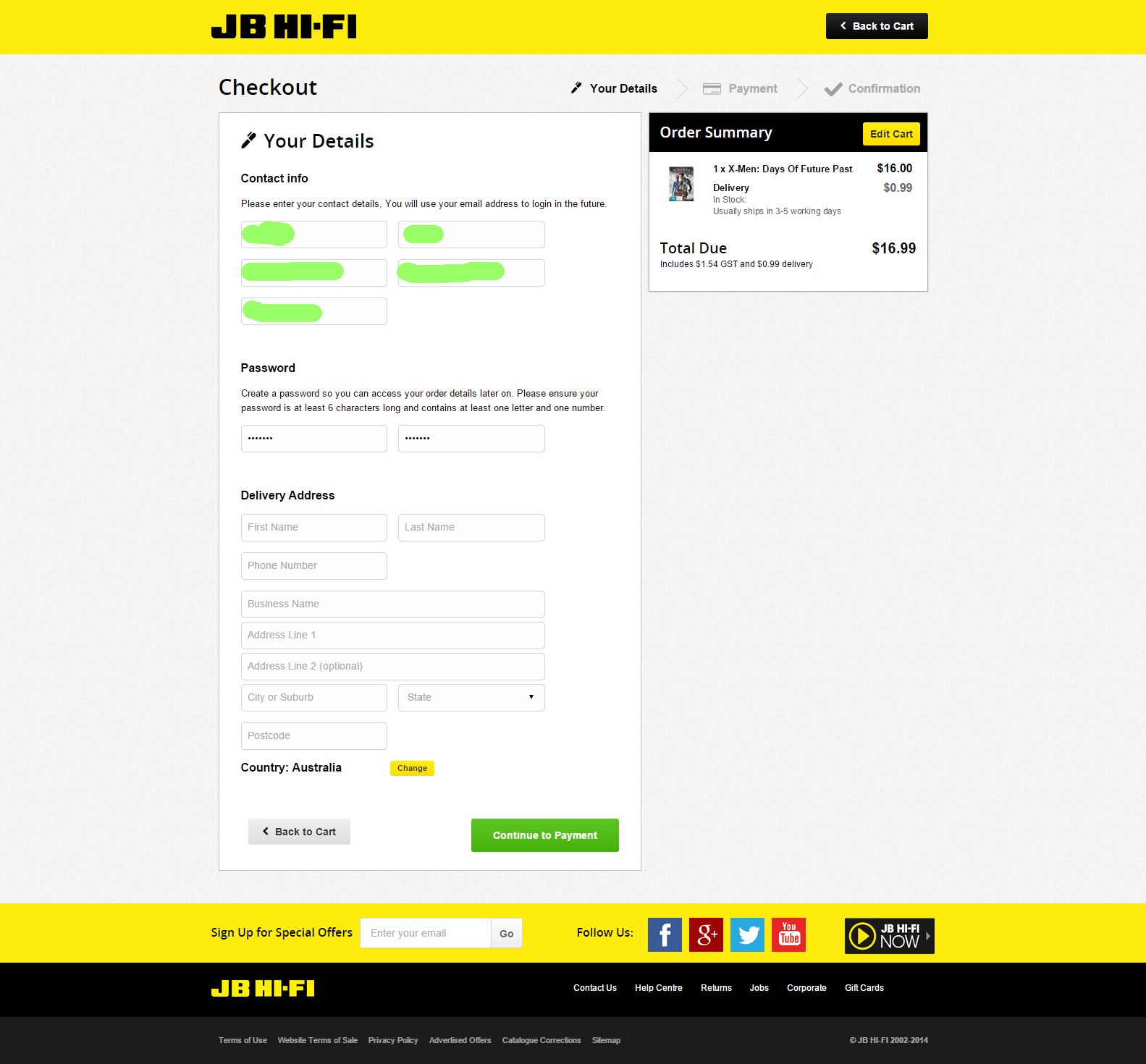The image showcases a checkout page from the JB Hi-Fi website, characterized by its distinct yellow and black color scheme. At the top, against a prominent yellow banner, the JB Hi-Fi logo is displayed in bold black letters. To the right of the logo, a black rectangle with white text reads "Back to Cart."

Beneath this section, a grey background sets the stage for the checkout process. The sequence "Checkout" is followed by steps listed as "Your Details," "Payment," and "Confirmation." Within the "Your Details" section, users are prompted to enter their contact information via five fields that are obscured by light green smudges. Below these fields, a section for creating a password is noted, with two masked entries indicated by dots.

Further down, the "Delivery Address" section includes empty fields for the first name, last name, phone number, and address details. The country is pre-set to "Australia," with an adjacent yellow rectangle labeled "Change." Users can navigate back to the cart or proceed by clicking "Continue to Payment."

On the right side of the page, an "Order Summary" rectangle provides detailed information about the purchase. It lists 1x "X-Men: Days of Future Past" priced at $16, with a note that the item is in stock and typically ships within 3-5 working days for an additional 99 cents. The total amount due is $16.99.

At the bottom of the page, another yellow banner offers a sign-up for special offers, accompanied by a white search bar and various social media icons (Facebook, Google Plus, Twitter, YouTube) under "Follow Us." A black rectangle labeled "JB Hi-Fi Now" sits above a black banner featuring links for "Contact Us," "Help Center," "Returns," "Jobs," "Corporate," and "Gift Cards," all in white letters. The very bottom of the page, against a grey banner, lists links to the "Terms of Use," "Website Terms of Sale," "Privacy Policy," "Advertised Offers," "Catalog Corrections," and the "Sitemap."